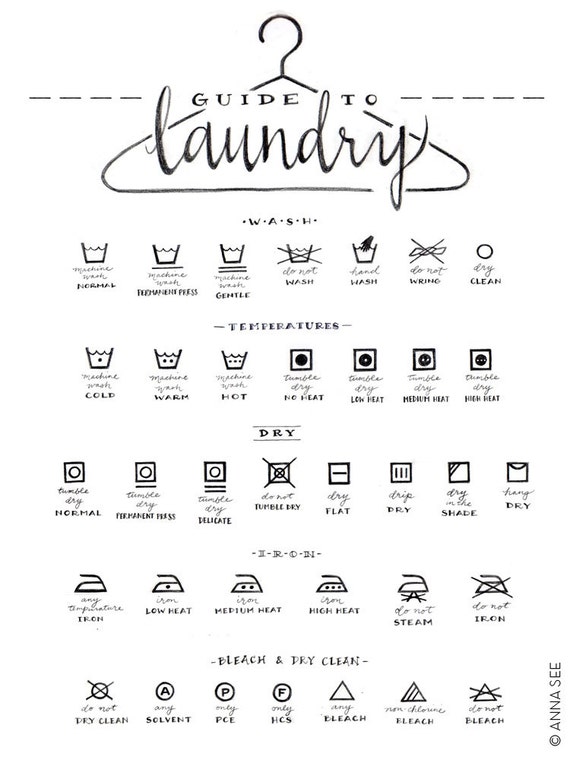This detailed and meticulously designed "Guide to Laundry" by artist Anna C, prominently features a black and white metal cloth hanger at the top, around which the title is artistically arranged with "GUIDE TO" in capital letters and "Laundry" in a script font. The graphic is sectioned into categories: Wash, Temperatures, Dry, Iron, and Bleach & Dry Clean. Ensuring clarity, each category is labeled in bold, black capital letters, accompanied by corresponding minimalistic icons, totaling roughly 30 to 40 symbols. These icons visually represent different settings, such as "Normal," "Gentle," and "Clean" under Wash, or "Cold," "Warm," and "Hot" under Temperatures. The drying methods include "Normal," "Permanent Press," "Delicate," among others, and are illustrated with various straightforward graphics like dots in a water bowl indicating temperature levels. Spanning five rows, this comprehensive guide not only covers washing cycles and temperatures but also ironing instructions and bleach/dry clean options. This functional and aesthetic piece aims to simplify laundry tasks through clean, minimalist visual cues, with a subtle watermark of the artist's name at the bottom right corner.